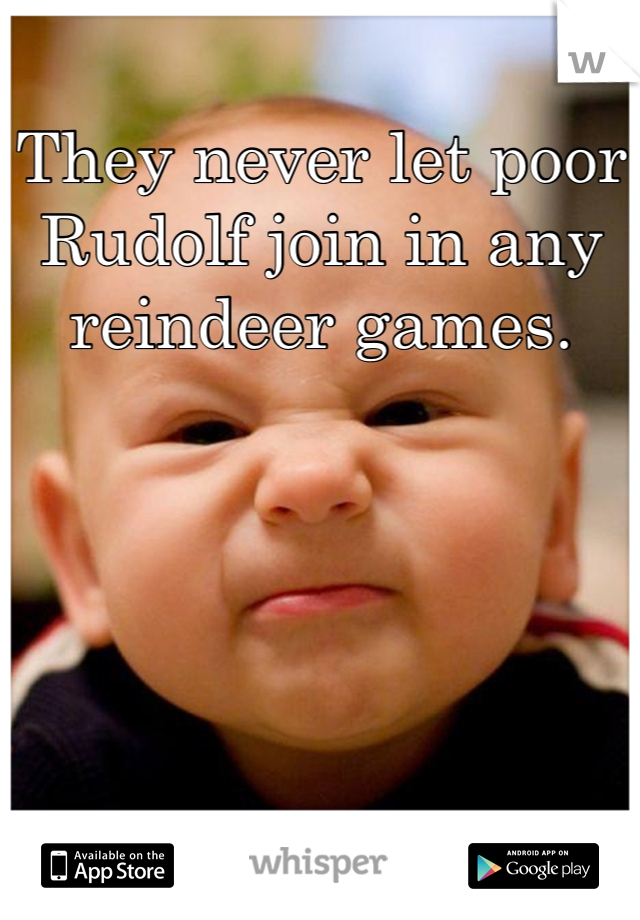The image is a screenshot of a meme taken from the Whisper app, which includes advertisements for the App Store and Google Play at the bottom. The central focus of the image is a baby with chubby cheeks and a scrunched-up face, looking directly at the camera. The baby’s expression mixes elements of playfulness and displeasure, with its nose crinkled and lips puckered. In white text, the meme humorously reads: "They never let poor Rudolph join in any reindeer games." The top right corner of the meme is folded down, revealing a small 'W' on the back. The background of the image is blurred, hinting at an indoor setting and offering no distinct details, allowing the baby and the text to stand out prominently.